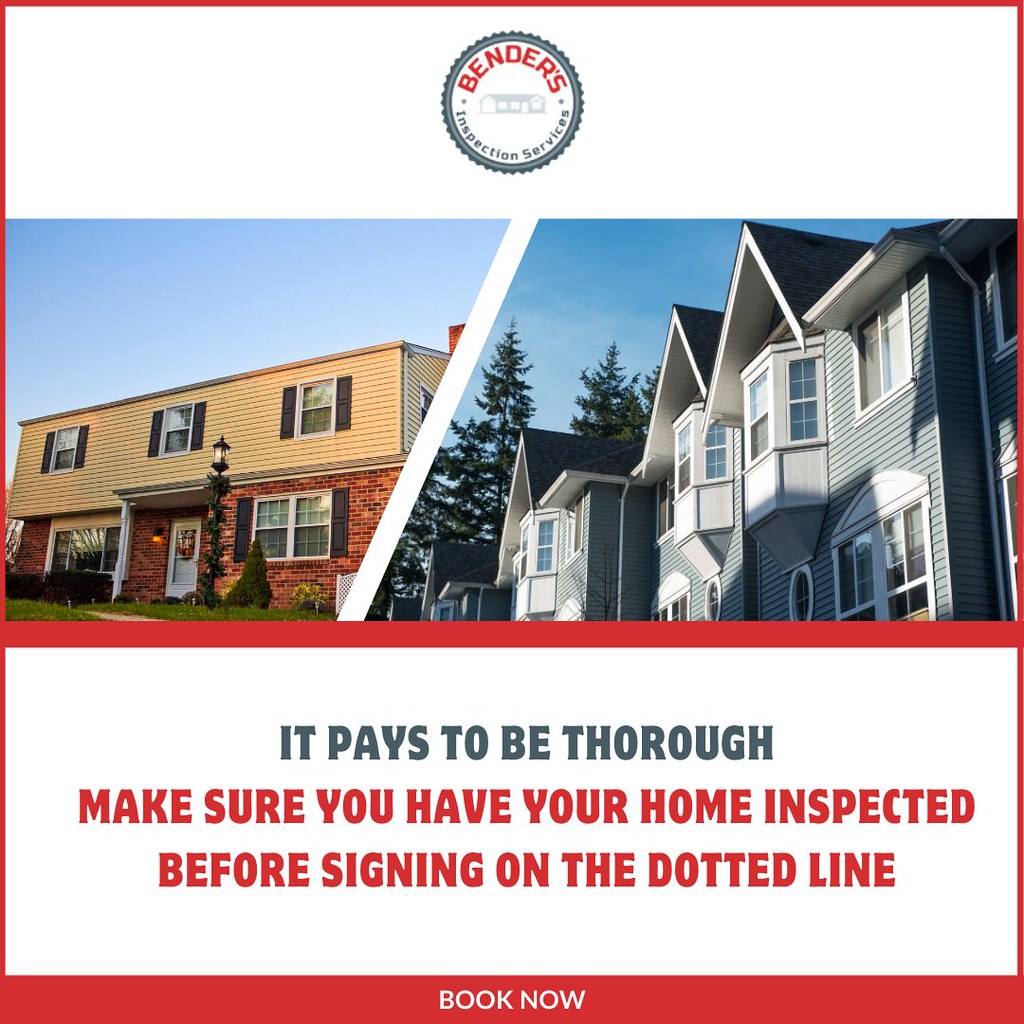This is a large, square advertisement for a home inspection company, Benders Inspection Services, framed by a red border. The top part features a solid white background with a central circular logo. The name "BENDERS" is prominently displayed at the top of the circle in red, all caps letters, while "INSPECTION SERVICES" is written at the bottom of the circle in black letters. Inside the circle is a drawing of a house.

Below this, the main section of the advertisement showcases two contrasting house images separated by a diagonal white line. On the left, there is a two-story, colonial-style house with a reddish-brown brick ground floor and brown-painted upper floor. It features a green lawn, black shutters, and a white door, under a clear blue sky. On the right, there are gray, two-story townhomes with bluish-gray paint and triangular, hipped roofs, accented by white trim around the windows and doors, set against a backdrop of tall pine trees and a blue sky.

The bottom section of the advertisement consists of a white rectangular background with the text "IT PAYS TO BE THOROUGH" in dark blue font. Below this, in red text, it says, "Make sure you have your home inspected before signing on the dotted line." The phrase "BOOK NOW" is prominently displayed in all caps white letters against the red border at the very bottom.